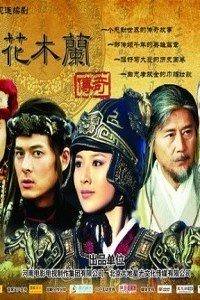The movie poster features a striking gold background with several lines of Asian characters at the top and more at the bottom. The bottom half showcases the profiles of three distinct individuals set against the golden backdrop. On the left, a man appears with an intense expression, donning a dark-colored metal headband and dark clothing, suggesting an aura of focus and determination. At the center is a woman exuding confidence, adorned in a heavily decorated bulbous metal helmet with gold trim. She wears a red collar and wide metal shoulder pads attached to black armor. To the right, an older man with a long beard, mustache, and grayish hair is depicted in gray robes, adding a sense of aged wisdom to the scene. Collectively, the characters give off an air of historical warriors or legendary figures, further emphasized by the elaborate and stylized attire.